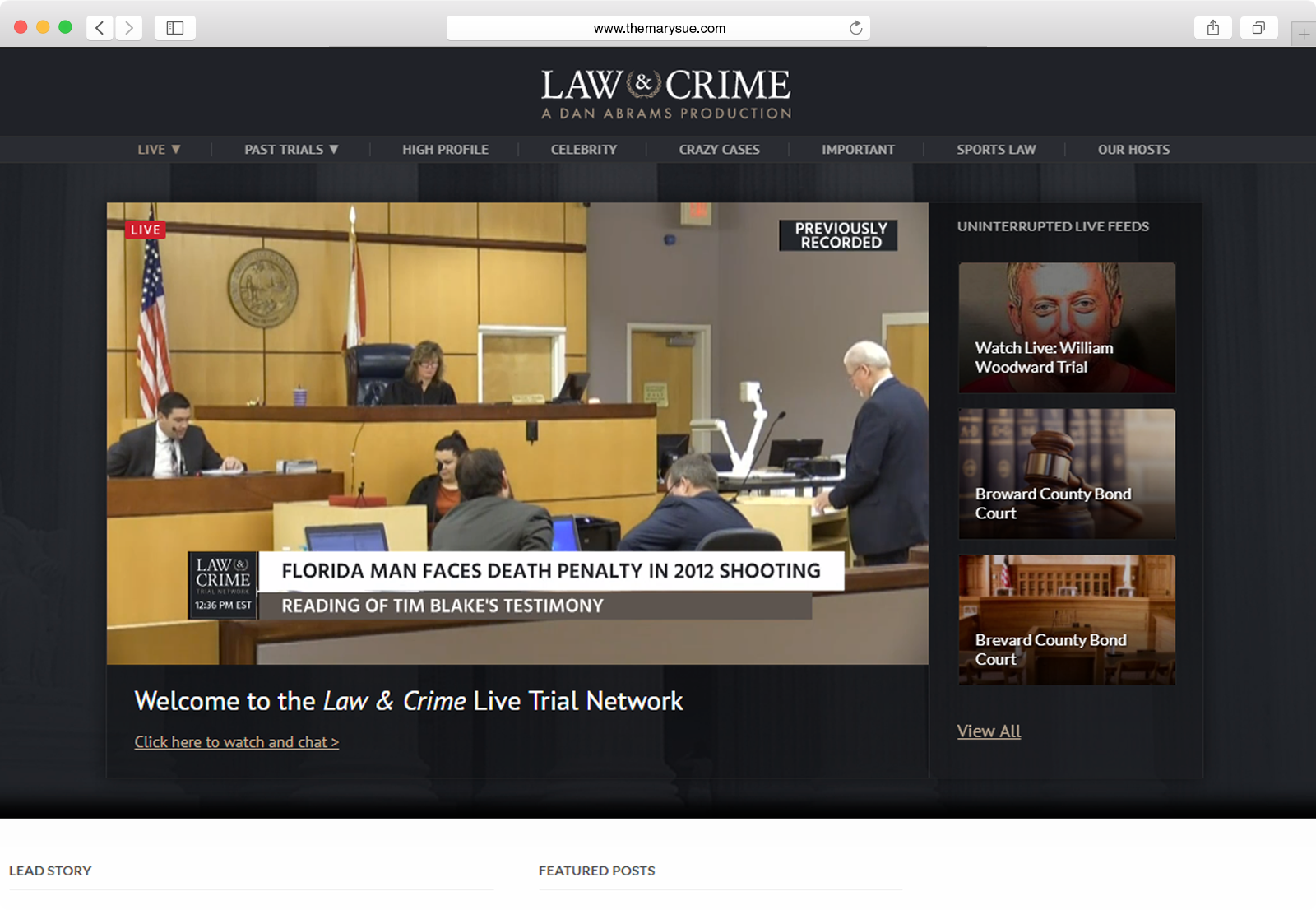The image depicts the homepage of a law office's website, specifically www.TheMarySue.com, featuring content related to "Law and Crime, a Dan Abrams production." 

In the upper left corner, three circles appear in red, orange, and green, likely representing browser window controls. Adjacent to these circles are left and right arrows for navigation.

Positioned at the top center is the URL, "www.TheMarySue.com." Directly beneath, the site's header displays "Law and Crime, a Dan Abrams production," followed by a navigation menu with several categories: "Live" (in light brown text), "Past Trials," "High Profile," "Celebrity," "Crazy Cases," "Important," "Sports Law," and "Our Posts."

Dominating the middle of the page is a large image of a courtroom scene. It features a female judge, a man standing to her side, and an audience of predominantly older individuals seated in the gallery.

To the right of the courtroom image, three distinct boxes provide additional information:
1. "Watch Live William Woodward Trial"
2. "Broward County Bail Court"
3. "Broward County Bond Court"

Each box offers quick access to live or recorded legal proceedings.